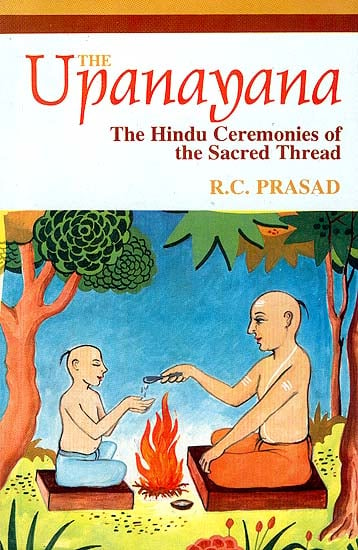The book cover titled "Upanayana: The Hindu Ceremonies of the Sacred Thread" by R.C. Prasad features an intricate, watercolor-style illustration. It depicts two Hindu figures sitting cross-legged on wooden blocks, engaged in a traditional ceremony. Both figures are shirtless, with a small tuft of hair in a ponytail at the back of their otherwise bald heads. The person on the right, an adult wearing red pants, holds a spoon over a ceremonial fire, dropping a substance—possibly water—into the open palms of the smaller figure on the left, who is wearing blue pants. The scene is set against a backdrop of a blue sky and lime green grass, with trees framing the image on both sides, suggesting a forest environment. The detailed illustration captures a moment of ritualistic significance amidst a serene natural setting.